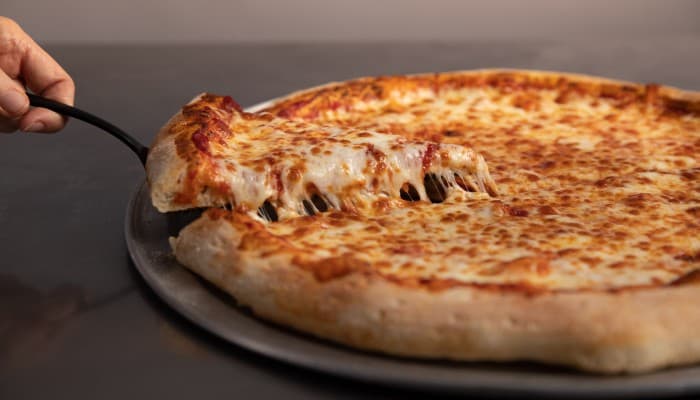The image captures a whole, round cheese pizza with a puffy, light brown crust and golden, bubbly cheese adorned with hints of browning on top. Positioned on a silver pizza tray, the pizza sits on a table with a black countertop in the background. From a side-angle perspective, you see a hand—specifically the thumb and index finger—holding a black utensil, lifting a single wedge-shaped slice of the pizza slightly above the rest, causing a gentle cheese pull. The focus is on the action of removing the slice, with both the lifted slice and the cheese pull being sharply in focus, while the far edges of the pizza and the background are softly blurred, giving a shallow depth-of-field effect. The simple backdrop draws full attention to the inviting, classic cheese pizza.